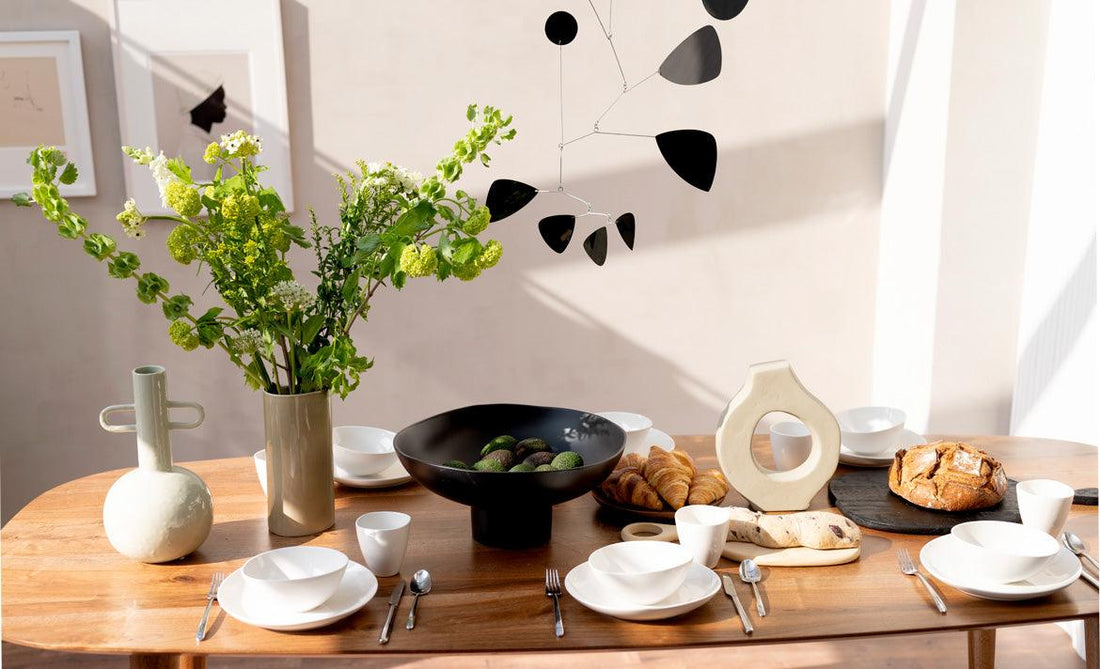The image depicts a high-quality, oval-shaped kitchen table prepared for breakfast. The wooden table with a subtle grain is elegantly set for six, featuring white plates, bowls, and mugs, each accompanied by a set of forks, knives, and spoons. In the center, a black ceramic bowl holds avocados, surrounded by a selection of pastries, including croissants. A large loaf of bread rests on a serving tray. The table is decorated with a variety of artistic ceramic pieces and an ornamental pot, possibly for pouring water, on the left. There is a vase with light green and green flowers adding a touch of nature. Overhead, a thin, silver, abstract mobile-like decoration with black weights creates an artistic flourish without providing lighting.